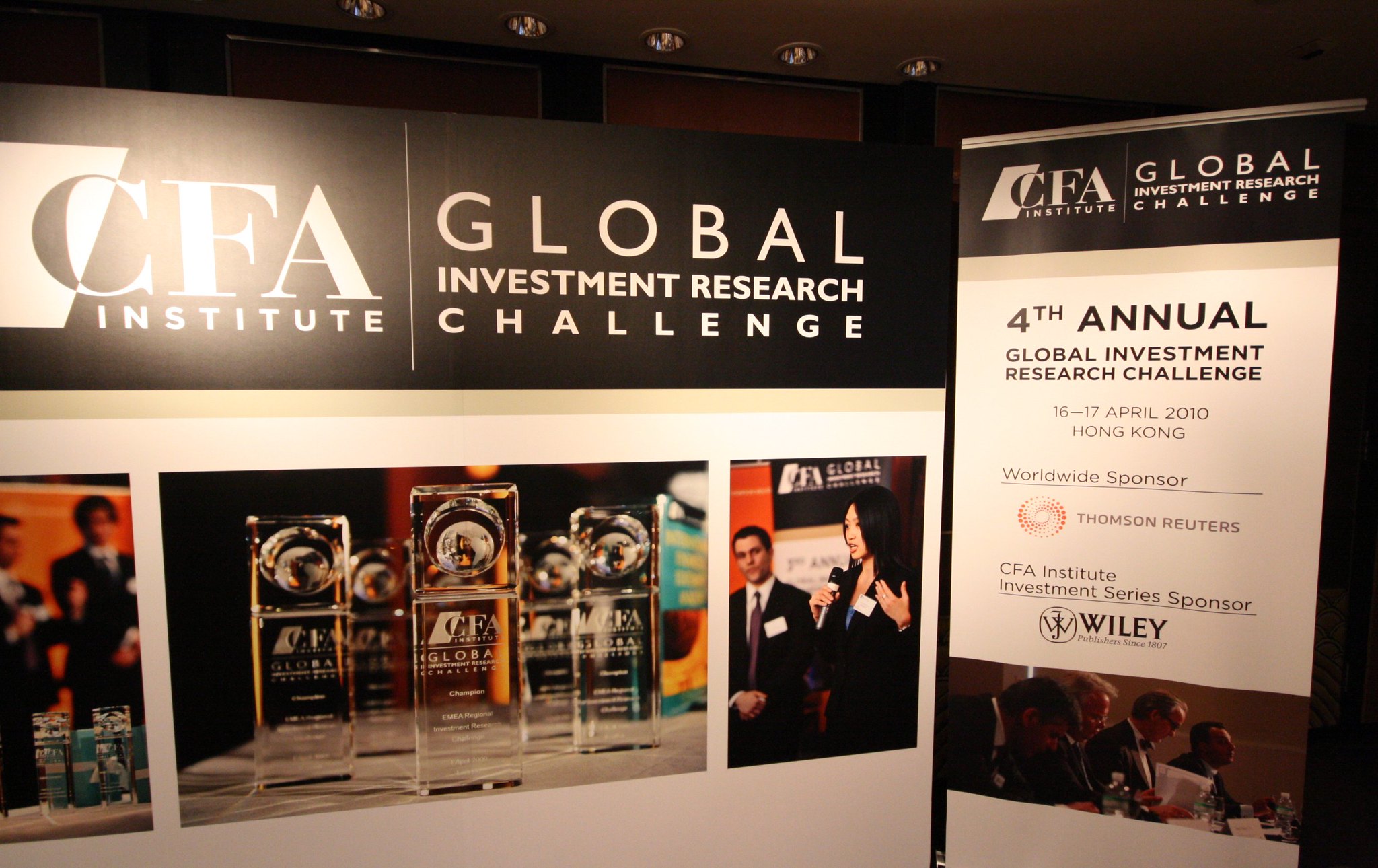Inside an event hall, illuminated by spotlights, two promotional banners stand side by side, presumably at the entrance or foyer of a convention or conference. The larger banner on the left is a wide, rectangular display with a black header that reads "CFA Institute Global Investment Research Challenge" in white text. Below the header, three images are presented: the central one depicting glass awards, while the flanking images include a photo of a formally dressed man and woman speaking into a microphone, and an out-of-focus shot of the awards again.

Adjacent to this, a taller, narrow rectangular banner mirrors the same black header with "CFA Institute Global Investment Research Challenge" text. Beneath this header, the banner details the "Fourth Annual Global Investment Research Challenge," highlighting the dates "16th, 17th of April, 2010" in Hong Kong. The sponsors listed include Thomson Reuters as the worldwide sponsor and Wiley as the CFA Institute Investment Series sponsor, all set against a white background. The banners collectively illustrate the prestige and sponsorship of the event, enhancing the formal ambiance of the interior space.